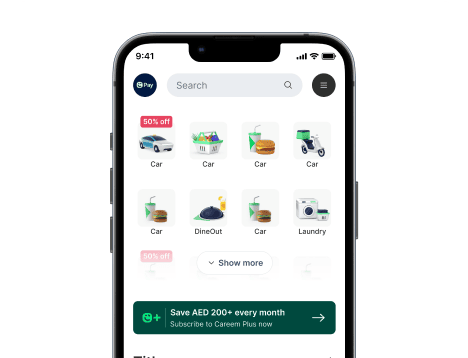The image depicts the interface of an ordering app displayed on an iPhone screen, complete with the phone's top status indicators showing the time as 9:41. The app's interface features a dark green circular icon labeled "Pay" at the top left corner. Centrally positioned to the right of this icon is a main search function symbolized by a magnifying glass. On the far right, there's a black circle containing a hamburger menu.

Beneath these icons, a prominent red rectangular banner displays a "50% off" promotion in bold white lettering. This banner overlays the category section, where multiple items are listed under the label "Car." The first item in the top row is an image of a sedan. The second item transitions from the car theme, depicting a grocery basket filled with various items. The third item, also labeled "Car," features an image of a cheeseburger and a drink with a straw, styled in white and green. The fourth item under "Car" shows a white scooter equipped with a green basket on the back.

Additional categories follow, including "Car Dine-out" and "Car Laundry," each with distinct logos. Below these categories, a dark green rectangular section promotes a subscription service with the text, "Save AED 200+ every month, subscribe to Kareem Plus now," accompanied by an arrow and a smiley face icon enhanced with a plus sign.